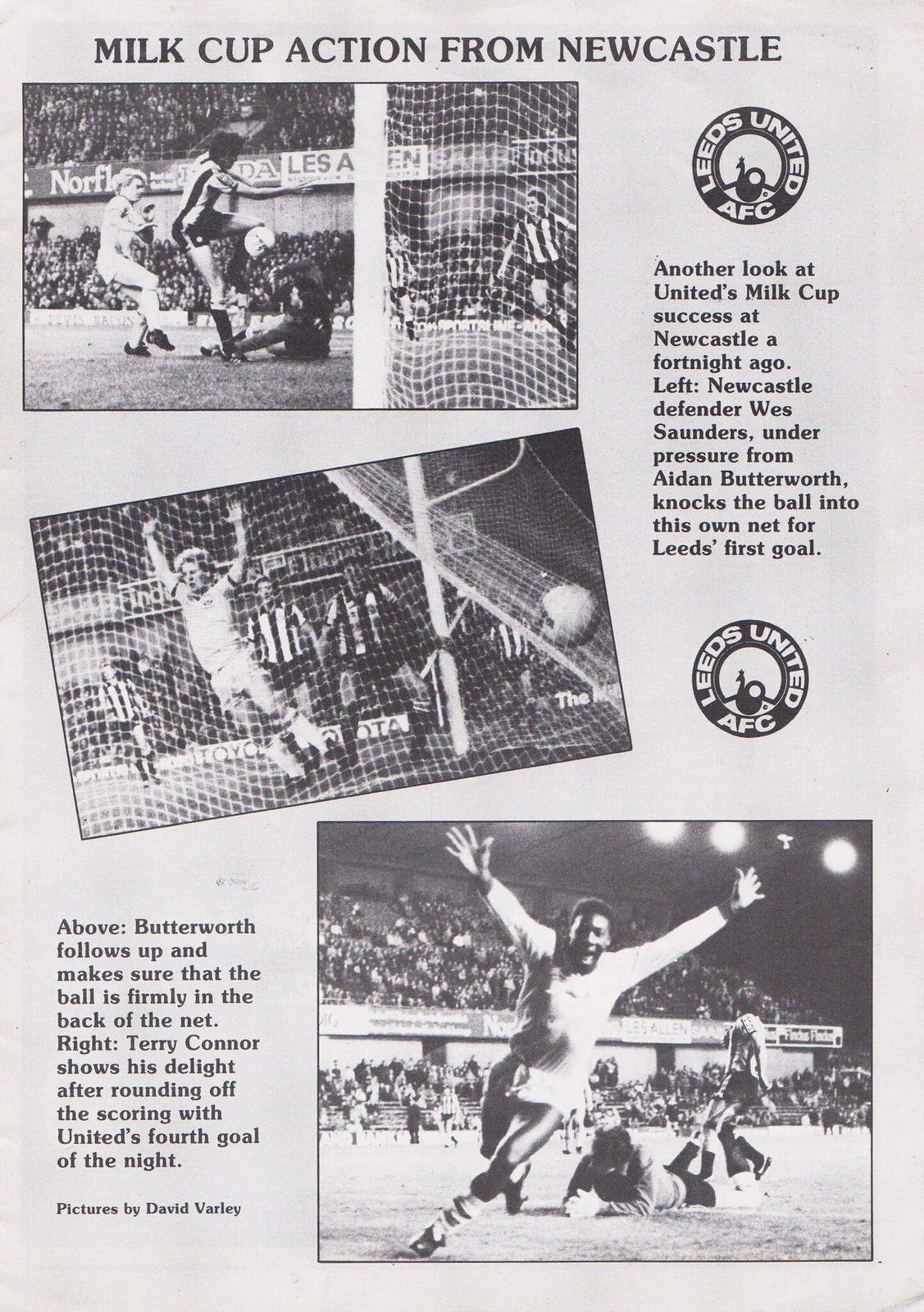The image is a scanned piece of paper, likely from an old magazine or program, depicted in black and white with details about a soccer match titled "Milk Cup Action from Newcastle" at the top in capital letters. Below the title, there's a description of Newcastle defender Wes Saunders, under pressure from Leeds United AFC's Aiden Butterworth, inadvertently knocking the ball into his own net for Leeds' first goal. An additional caption recounts Butterworth ensuring the ball is in the net and Terry Connor celebrating after scoring United's fourth goal of the night. The visuals include photographs by David Varley: one showing players in action on the field with a soccer ball and net, another capturing a player who has just scored, and an image of a jubilant player celebrating with raised hands.